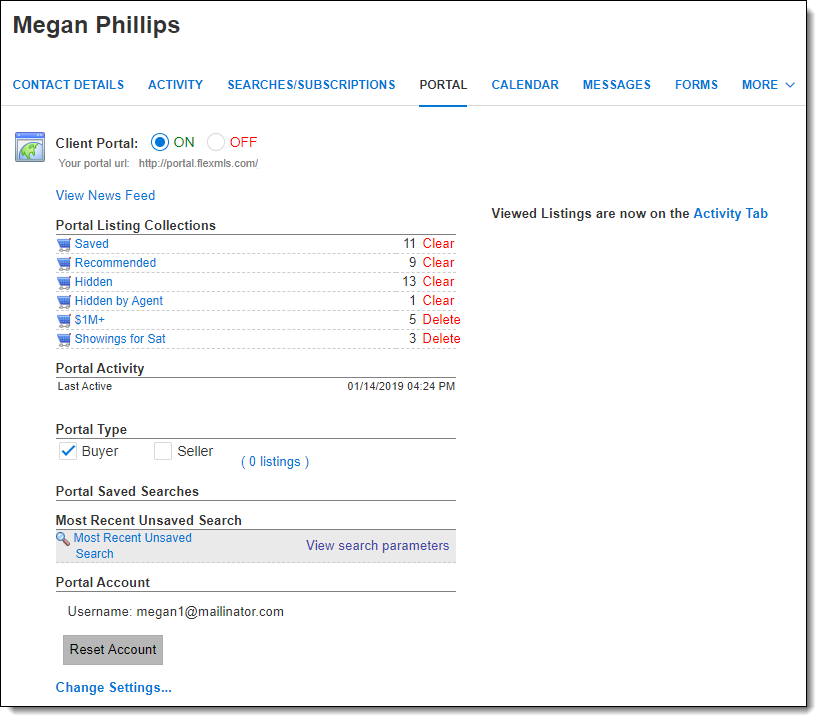This image is a detailed screenshot set against a white background with thin gray lines marking its edges. In the upper left corner, the name "Megan Phillips" is displayed in dark, bold black print. Below her name is a horizontal line of navigation options in blue text, listing: "Contact Details," "Activity," "Searches and Subscriptions," and "Portal," which is underlined, followed by "Calendar," "Messages," "Forms," and a dropdown menu indicated by "More." 

Directly beneath these options, we see the section labeled "Client Portal" with a toggle switch to the right. The switch is set to "On," which is circled and highlighted in blue. Below the toggle switch, the text "Your portal URL: http://portal.flexmls.com" is displayed. An informative note reads, "Viewed listings are now on the activity tab."

Further down, a prompt labeled "View News Feed" is visible. Next to it, there is a section with shopping cart icons, followed by several options: "Saved," "Recommended," "Hidden," "Hidden by Agent," "One Million Plus," and "Showings for Saturday." At the bottom, the "Portal Activity" section shows the last active date and time: "1-14-2019, 4:24 PM."